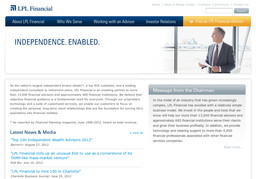A screenshot depicting a page from the LPL Financial website, characterized by an all-white background. At the top left corner, "LPL Financial" is displayed in blue text, accompanying the tagline "Independence Enabled." Adjacent to the title is an image of a man in professional attire – a business suit, tie, and white collared shirt – holding a paper and gazing to the left. Below the tagline are various paragraphs likely outlining the services offered by LPL Financial, although the text is small and difficult to read. In the bottom left-hand corner, clickable links are present, distinguishable by their transition from a dark black color to light blue. At the very top of the page, in the right-hand corner, is a small search bar with an accompanying search icon.